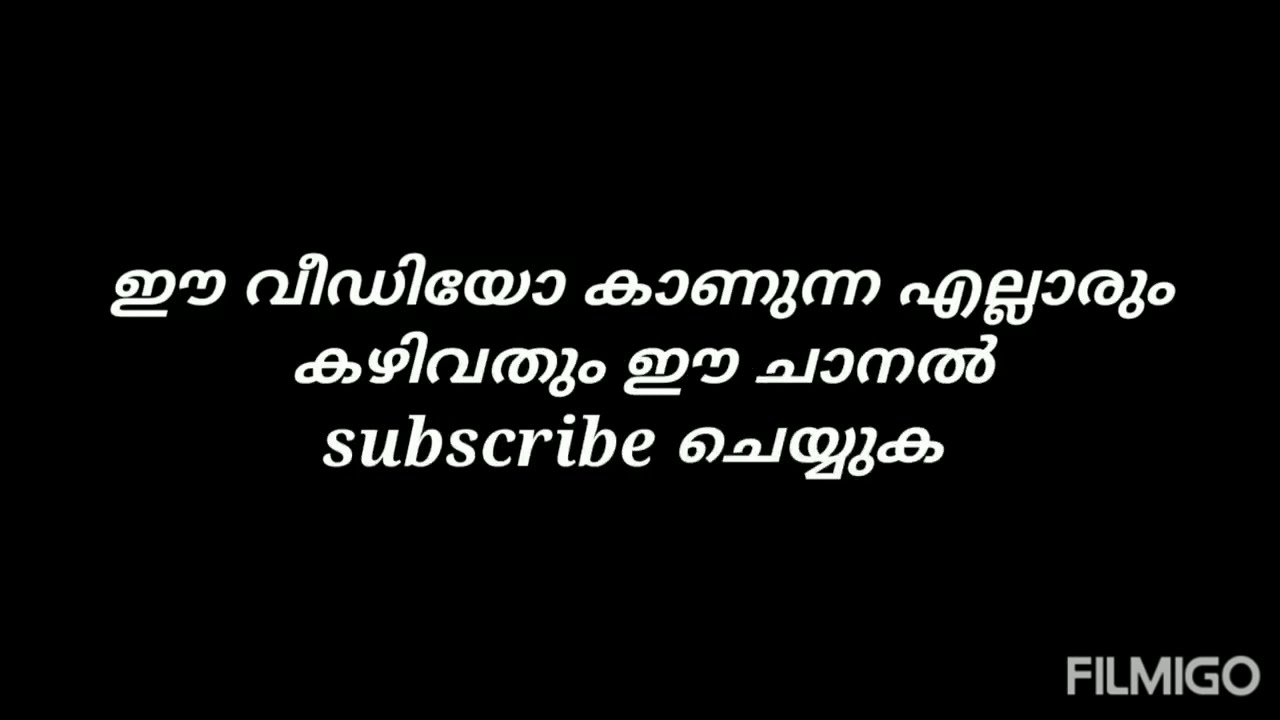The image features a matte black background with three lines of white text in the center, predominantly in a foreign language, likely Hindi. The top line is the longest, comprised of four words; the second line is slightly shorter with three words; and the third line is the shortest, starting with the English word "SUBSCRIBE" followed by a foreign term. In the bottom right-hand corner, "FILMIGO" is written in grey uppercase letters. The black background is pure and unadorned, and the image is shaped as a wide rectangle, approximately 1.5 times longer in width than its height. The overall arrangement of the text is centrally aligned against the stark black, creating a sharp contrast.